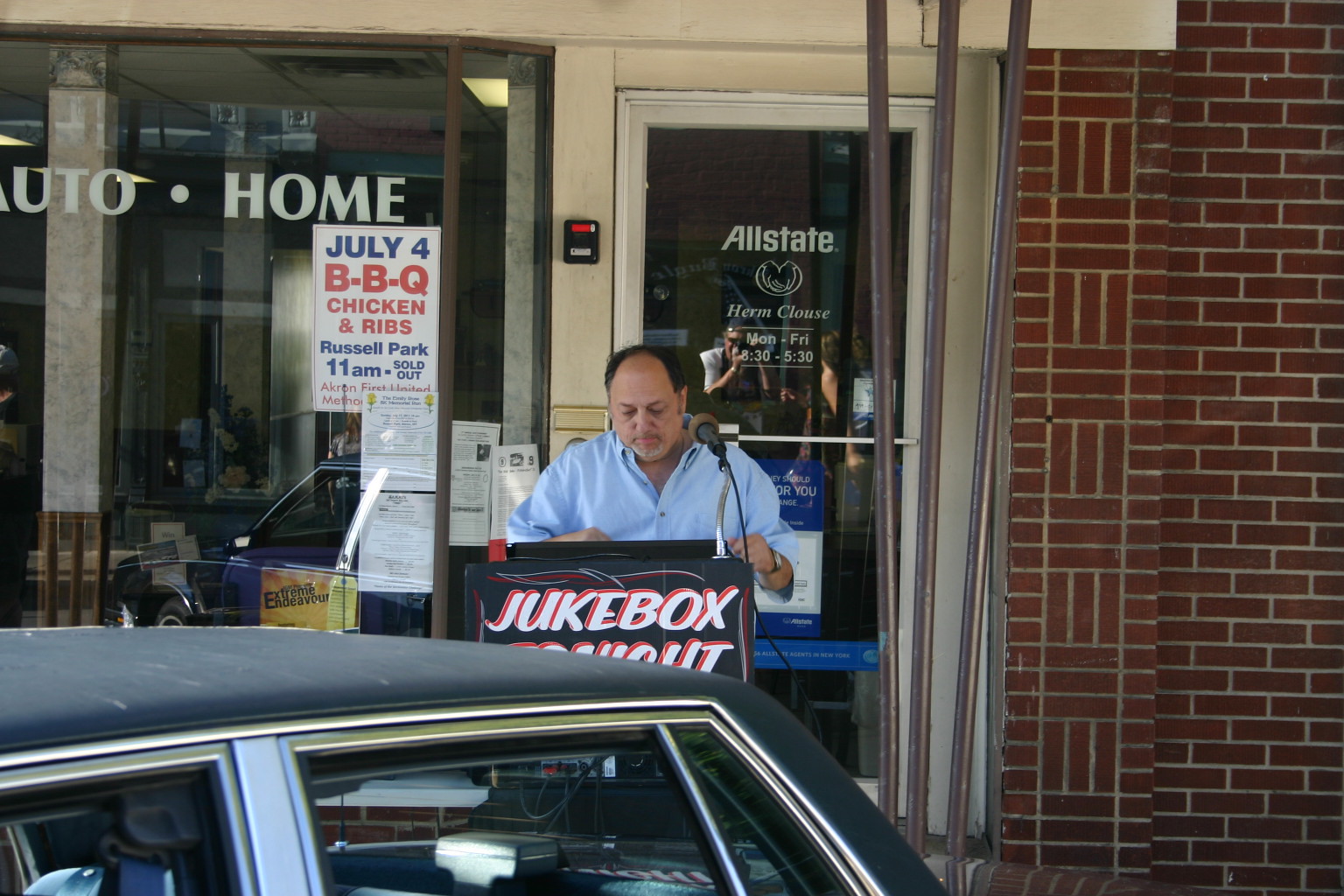In this image, taken outdoors in the middle of the day, we see a man standing at a microphone in front of a podium. The podium prominently displays white text with a red outline that reads "jukebox," with some obscured text beneath it. The man is centrally positioned within the scene and appears to be delivering a speech or announcement. Directly behind him, there's a building with a glass storefront door framed in metal, which bears the text "Allstate." The building features a red brick wall with an intricate design. Hanging on one of the storefront windows is a sign detailing a "July 4th BBQ, Chicken and Ribs at Russell Park, 11 a.m." In the bottom left corner of the image, the top of a parked car is visible. The overall color scheme includes dark blue, silver, black, red, orange, yellow, brown, tan, and off-white.